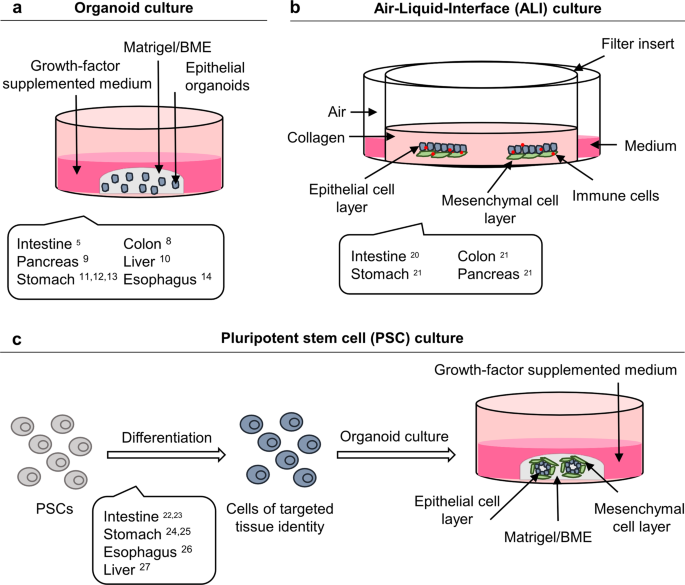In this detailed diagram, we observe a comprehensive overview of various cell culture techniques and their components, color-coded with black text, pink, blue, and green hues for clarity. At the very top, from left to right, the terms "organotypic culture" and "air-liquid interface culture" are prominently labeled, setting the context for the depicted methodologies.

Below, the diagram illustrates a container showcasing cultured items or cells. The container is detailed with annotations such as "growth factor-supplemented medium," "Matrigel," "epithelial organoids," "filter insert," "immune cells," "air," "collagen," and specific organs, including the intestine, stomach, colon, and pancreas. These labels indicate the intricate arrangement and the components involved in the culture process.

At the bottom, a distinct section is labeled with black text describing "pluripotent stem cell (PSC) culture." This part of the diagram shows PSCs transitioning, denoted by an arrow, to cells with a targeted tissue identity. To the right, the "growth factor-supplemented medium" is illustrated, pointing toward the differentiation into the epithelial cell layer and the mesenchymal cell layer, emphasizing the developmental process and differentiation facilitated by the growth factors.